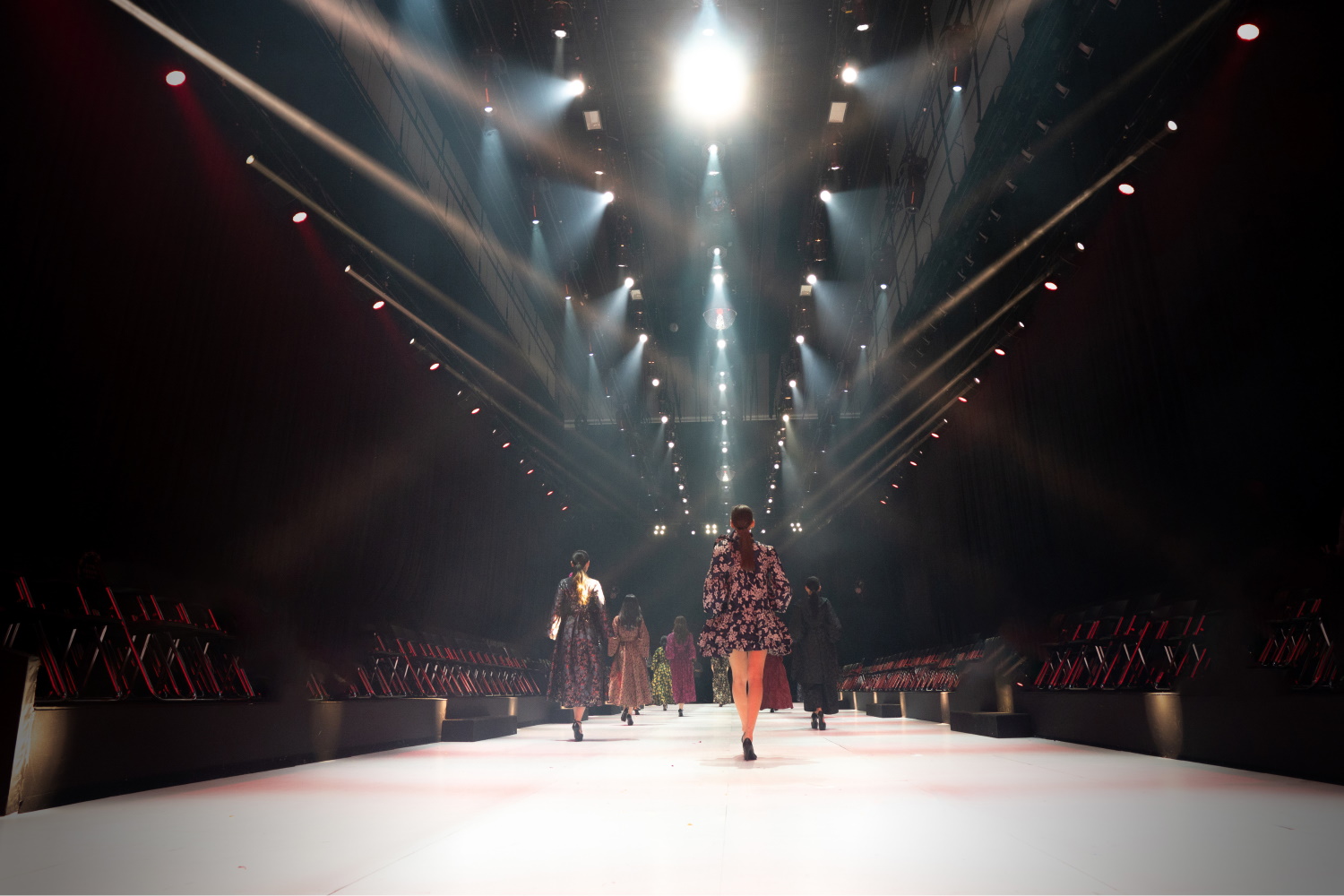This photo captures a long runway stage set in an interior space, illuminated by rows of bright overhead lights. The runway is white or cream-colored, and along its left and right sides are empty seats in black and red. Several models are seen walking away from the camera, practicing their walks. The models, all with long hair, are dressed in a variety of outfits including long dresses, cocktail dresses, and some with floral patterns. One model wears a purple dress, another has tights, and some are seen in black boots or shoes. The lighting makes the stage very bright, emphasizing the length and spaciousness of the venue, although no audience members are present in the stands.